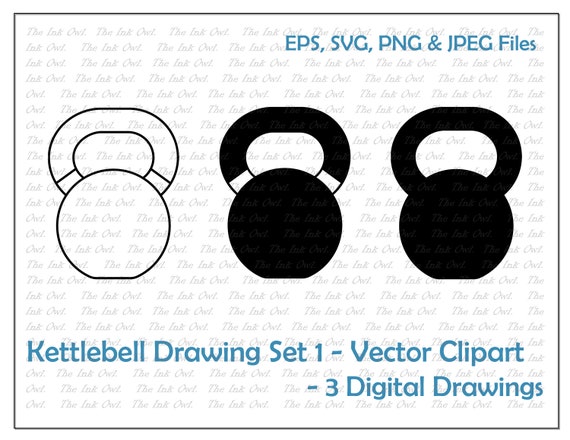The image is a graphic slide featuring three kettlebells set against a white background. The kettlebells are displayed from left to right: the first one is entirely white except for black outlines, the middle one is predominantly black with a small white section, and the right one is completely black. Across the top of the image, in blue text, it reads "EPS, SVG, PNG, and JPEG files." At the bottom, also in blue but in slightly larger text, it says "kettlebell drawing set one, vector clip art, three digital drawings." Throughout the entire image is a watermark that reads "The Ink Owl," likely indicating the creator and seller of these graphic designs.